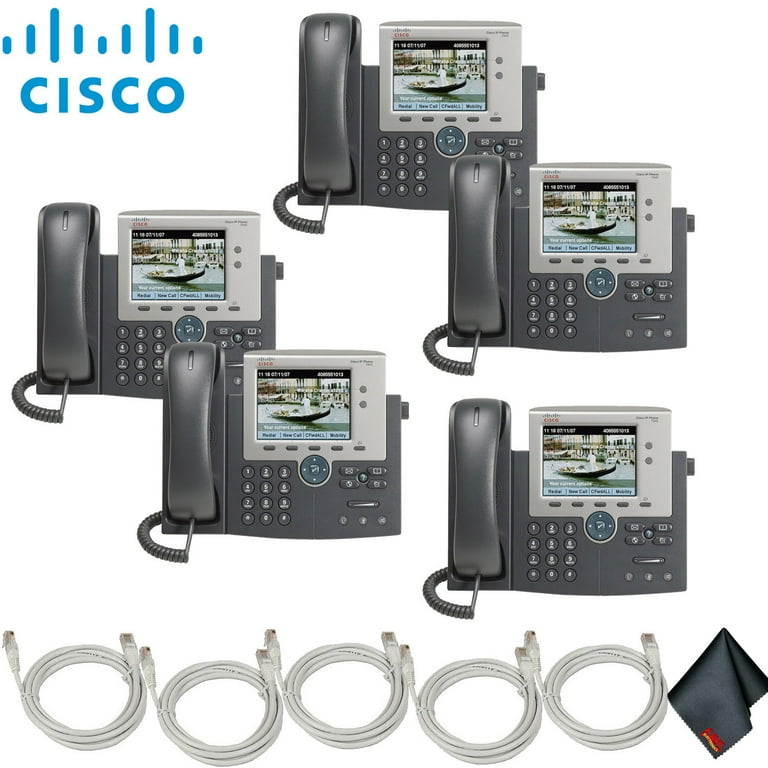The image intricately displays a series of five identical, corded office phones by Cisco, clearly highlighted by the distinct "CISCO" logo in blue at the top left corner with vertical blue bars above the letters. Each phone features a dark gray handset and buttons, accompanied by various function keys like voicemail and volume on the right side of the keypad. These phones boast built-in screens framed with a light gray bezel, each screen typically showing options like “new call” and a detailed image of a person standing on a small boat atop a body of water. Below the phones are five neatly coiled Ethernet cables and a folded cleaning wipe in black and red. The photograph captures the products with high clarity under bright and clear lighting, emphasizing the advanced functionality and design aimed at modern, professional settings.